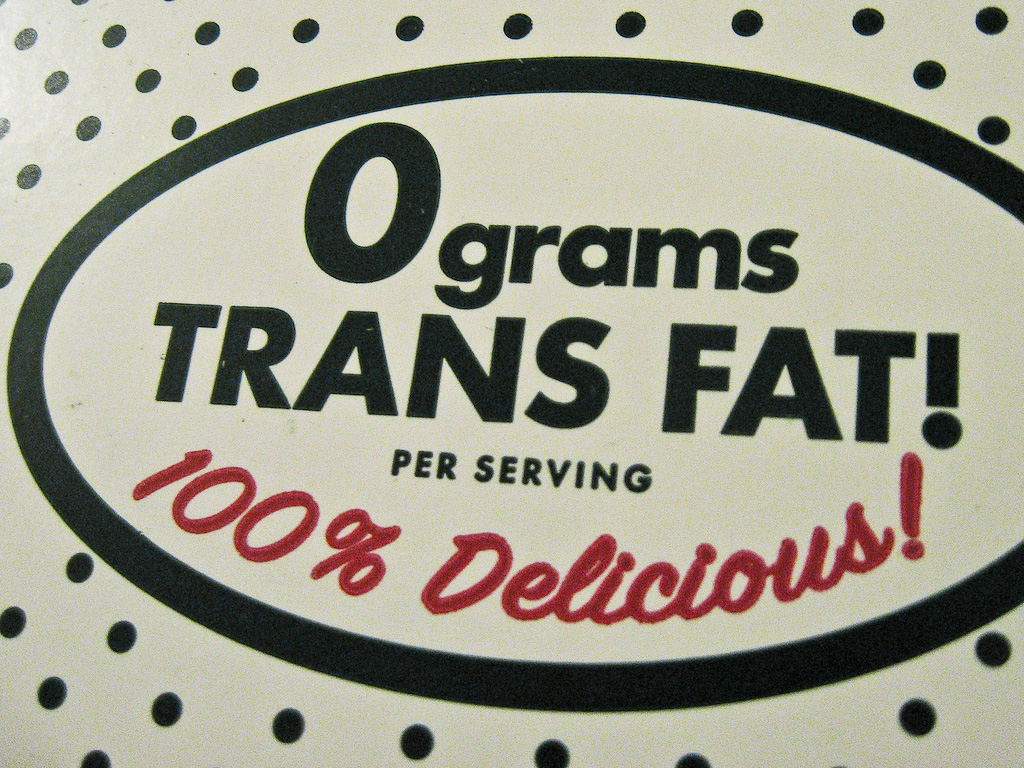This is a color photograph featuring an extreme close-up of a section of a food container. Central to the image is an oval-shaped label adorned with various texts. The prominent text within the oval reads "Zero grams trans fat" in bold black letters, followed by a smaller inscription underneath stating "per serving." Adding a touch of flair, the phrase "100% delicious!" is emblazoned in a bright red, fancier font towards the bottom of the label. Surrounding the oval are black and white spots, reminiscent of a classic Krispy Kreme box design, though the green typically associated with Krispy Kreme appears darker in this close-up. The detailed text and graphical elements on the oval label offer a mix of nutritional information, promotional text, and aesthetic design, captured in this tightly-framed shot.